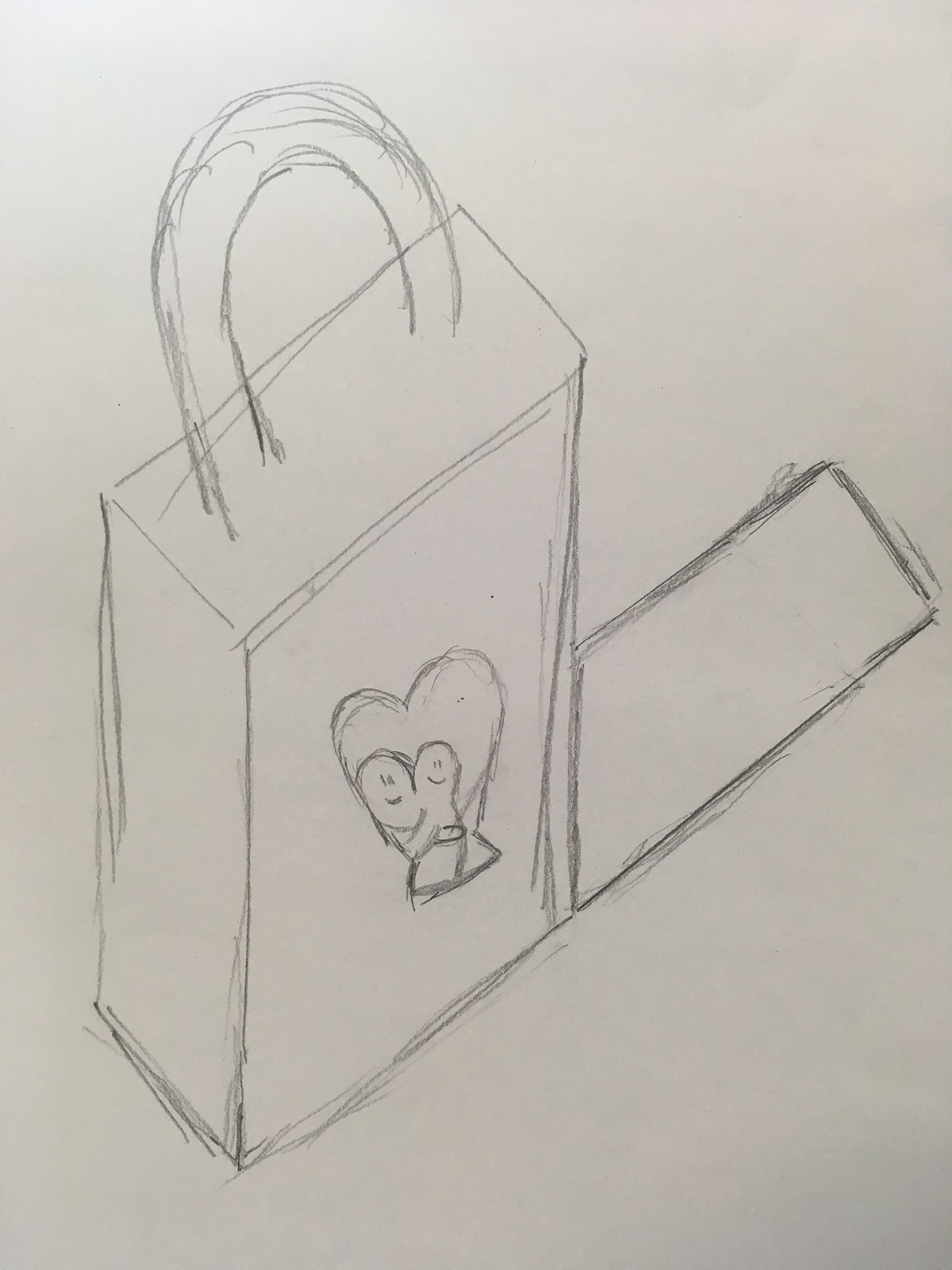This charming, hand-drawn image features a simple yet endearing depiction of a teapot, likely crafted by a child. The teapot, rendered in pencil on a white sheet of paper, showcases a thick handle and a moderate size. Uncolored and simplistic, the drawing gains its warmth from the details at its center: a large heart and a joyful stick-figure duo. The two smiling figures, possibly depicting friends or ladies, appear to be hugging, their hair subtly indicated. The teapot's 3D-like appearance adds a touch of depth to this delightful piece of art.